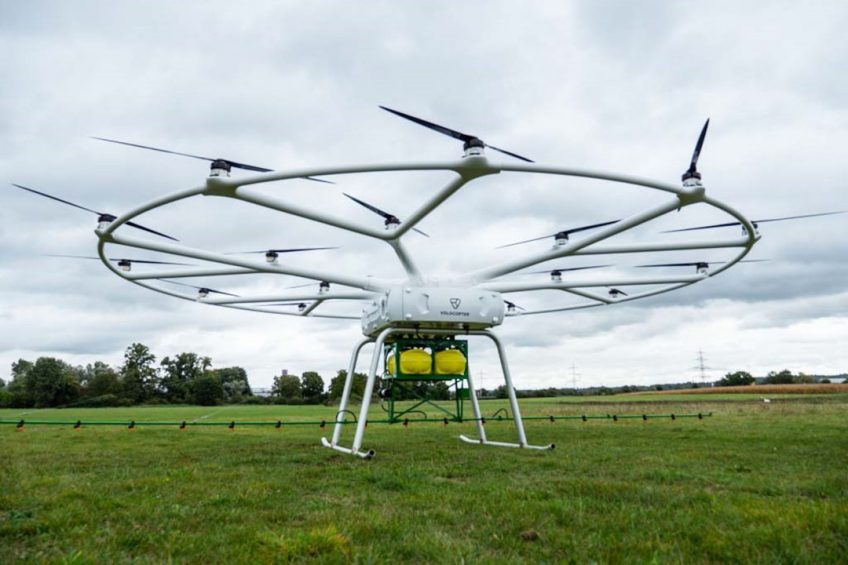The photograph captures a volocopter-style drone, predominantly white in color, stationed in a lush green field intended for irrigation. The drone features a prominent circular frame at the top, equipped with numerous black helicopter-style blades, suggesting its capacity for rotational lift. This frame is connected to the central body of the drone through multiple metal rods, providing structural integrity. The body of the drone consists of a metallic square section, beneath which a green cage structure houses yellow cylinders or containers. Additionally, green pipes or a long rod extend from the bottom, hinting at a watering or spraying function. The drone rests on two sturdy leg stands composed of metal rods. Surrounding the drone, the field exhibits an active sprinkler system, and in the background, a line of trees and power lines is visible under a cloudy, threatening sky that suggests impending rain.